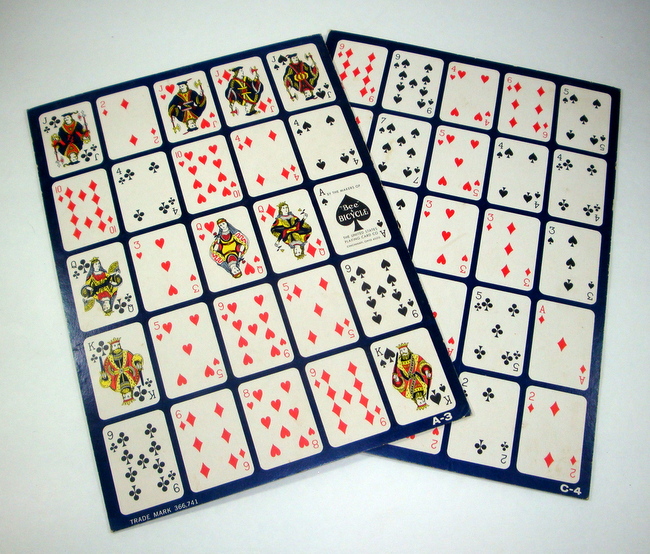This photograph captures two rectangular objects placed against a white surface with slightly darkened corners. The primary object on the left appears to be a piece of cardboard or possibly part of a board game, featuring a detailed 5x5 grid of playing cards. 

The cards on the grid are arranged as follows:
- Top row: Jack of Spades, Two of Diamonds, Jack of Hearts, Jack of Diamonds, Jack of Spades.
- Second row: Ten of Diamonds, Four of Spades, Ten of Hearts, Four of Diamonds, Four of Spades.
- Third row: Queen of Clubs (mistakenly referred to as "clover"), Three of Hearts, Queen of Hearts, Queen of Diamonds, Ace of Spades.
- Fourth row: King of Clubs, Five of Hearts, Nine of Hearts, Five of Diamonds, Nine of Spades.
- Fifth row: Jack of Clubs, Four of Hearts, Six of Diamonds, Five of Spades, Nine of Diamonds.

The first board partially overlaps another similar board beneath it. This secondary board displays another 5x5 grid, though the cards are not fully visible due to the overlapping. The visible top row includes: Nine of Diamonds, Nine of Spades, Four of Hearts, Six of Diamonds, and Five of Spades.

The first board features the text "A-3, trademark 366741" at its bottom edge, and the second board displays "C-4" in white on its bottom right corner. Both boards are primarily black or very dark blue and showcase standard playing cards with typical suits and colors. The "Bicycle" logo, synonymous with classic playing cards, is visible, suggesting these boards might be engaging tools similar to Lotería, but utilizing traditional playing card imagery.